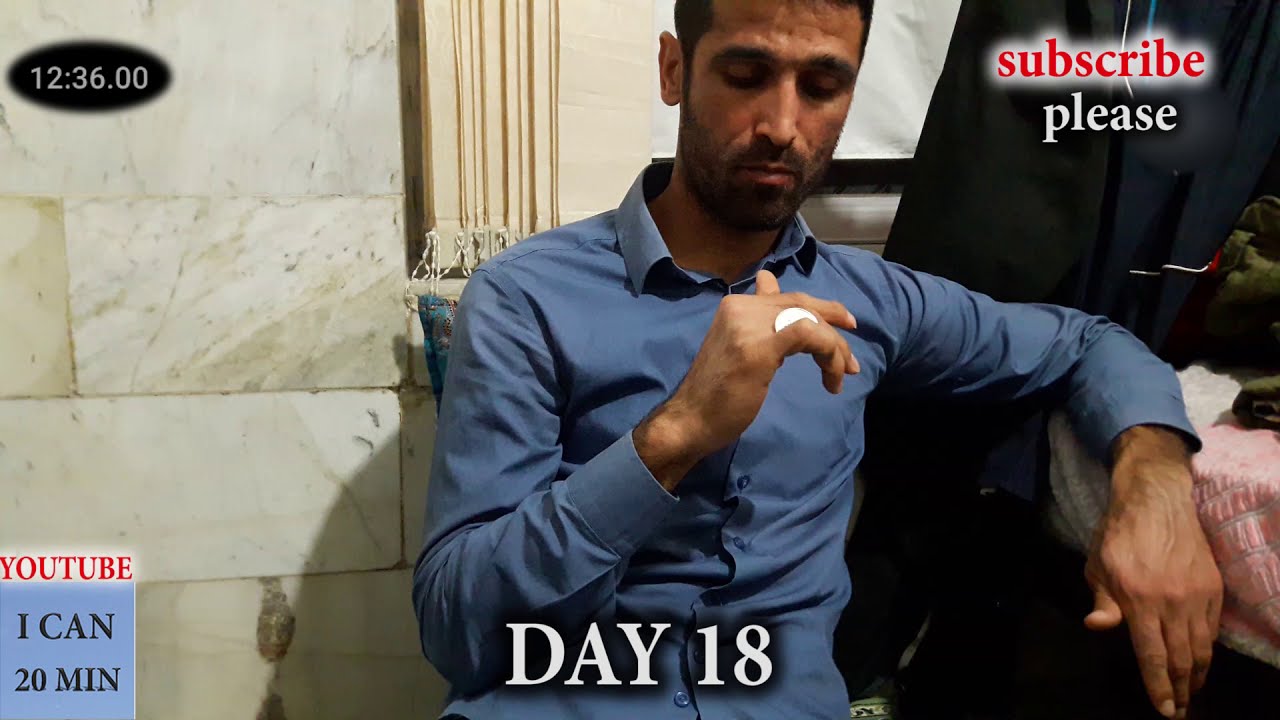A man of possible Arab or Indian descent sits in a room adorned with a cream-colored marble wall and some molding. He wears a blue long-sleeved button-up shirt and has short black hair with a trimmed beard. With his eyes closed, he appears to be concentrating, holding a white object or coin between his fingers of his right hand. The setting includes a pink table and a black curtain. The image contains several annotations: in the upper left corner, a time counter reads "12:36:00" set against a horizontally placed black oval background; in the upper right corner, "Subscribe please" is written, with "Subscribe" in red surrounded by a white glow and "please" in white; in the bottom middle, the text "Day 18" is displayed; and at the bottom left, it reads "YouTube I can 20 minutes." The overall color palette includes blue, white, tan, black, red, pink, and various shades of brown. The scenario hints at an intense focus, possibly on a game or task involving the coin.